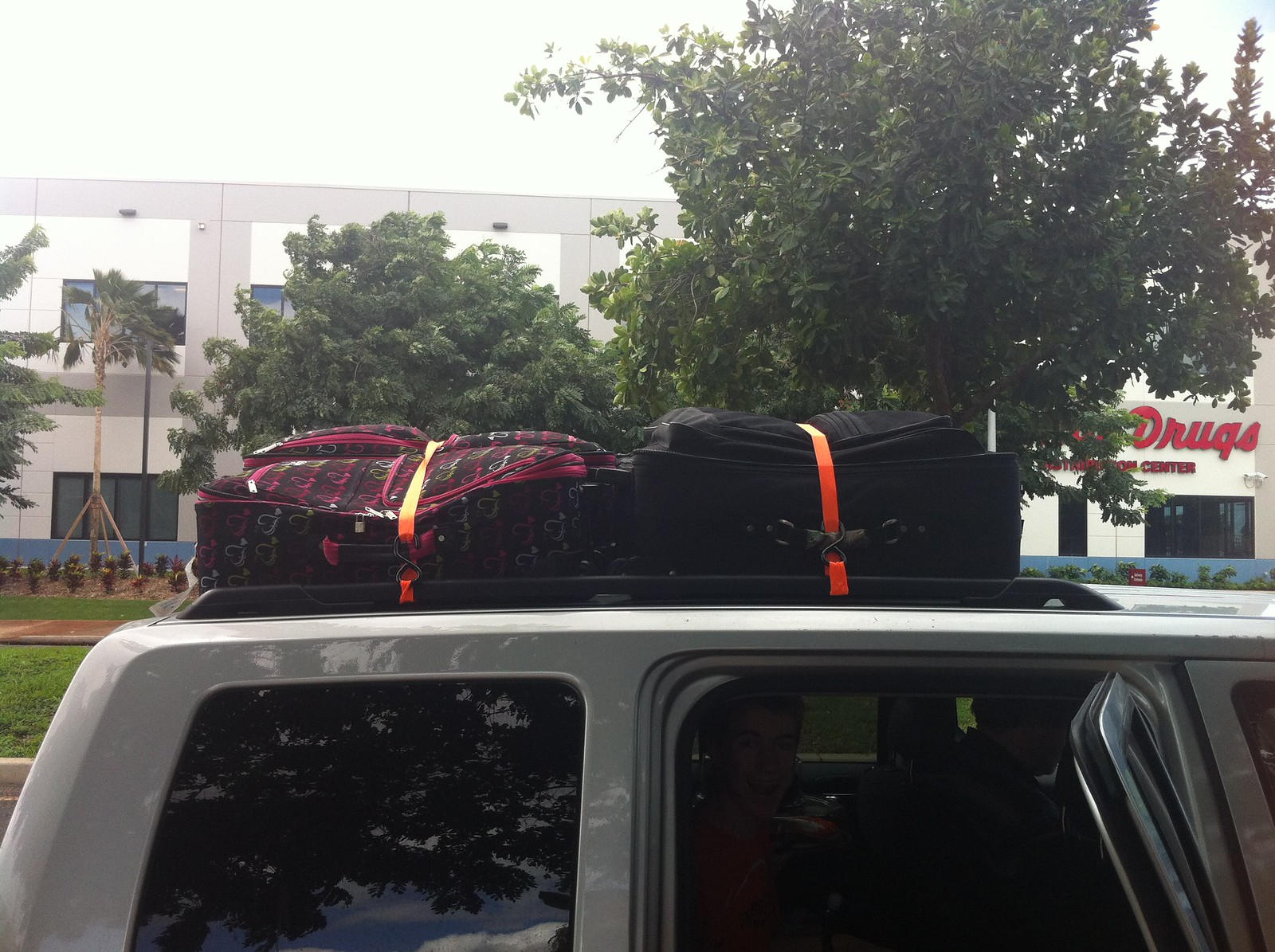This image depicts the top half of a gray SUV with darkly tinted windows and an open rear side door, where the silhouette of the driver is visible through the dark interior. Attached to the black roof rack are two large suitcases secured with bright neon orange straps that stand out vividly. The suitcase on the left features a black and pink heart pattern, while the suitcase on the right is a standard black fabric. The SUV is parked in a shopping district, flanked by two leafy green trees that obscure much of the background. Among the partially visible elements behind the trees, there is a sign with the word "drugs" in red script font, likely indicating a drugstore or a related business. Above this, the sky appears largely white, indicating daylight. The background also includes hints of large buildings and a clear blue sky.